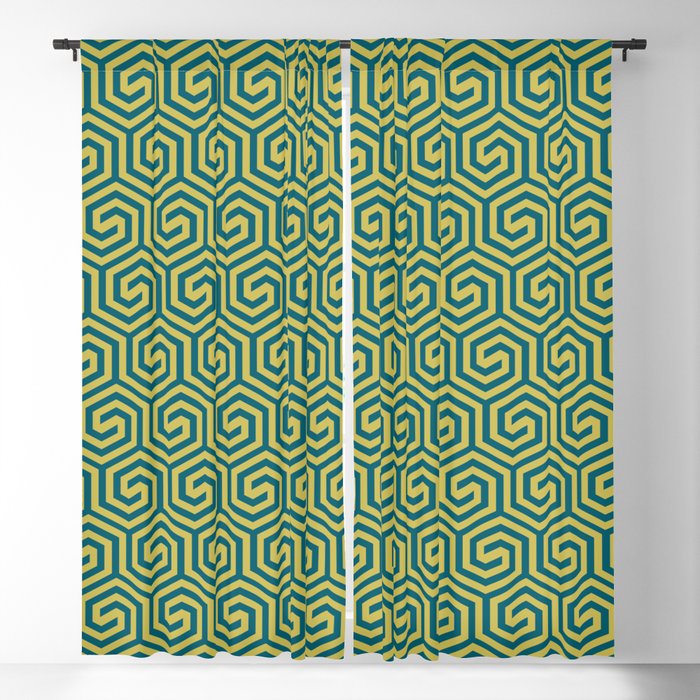The image depicts a product photo of a pair of plain, vertically hung curtains set against a white background. The curtains feature a repetitive geometric design with hexagonal shapes that swirl hypnotically into the middle, reminiscent of an Escher painting. The pattern consists of alternating lines of green and yellow, although some describe the colors as teal blue and light olive green. These colors create a somewhat unappealing aesthetic. The curtains are hung from a simple, straight wrought iron curtain rod, and they are parted slightly in the middle, allowing light to filter through. The overall look is minimalist with a focus on the unique, interlocking pattern of the curtains.